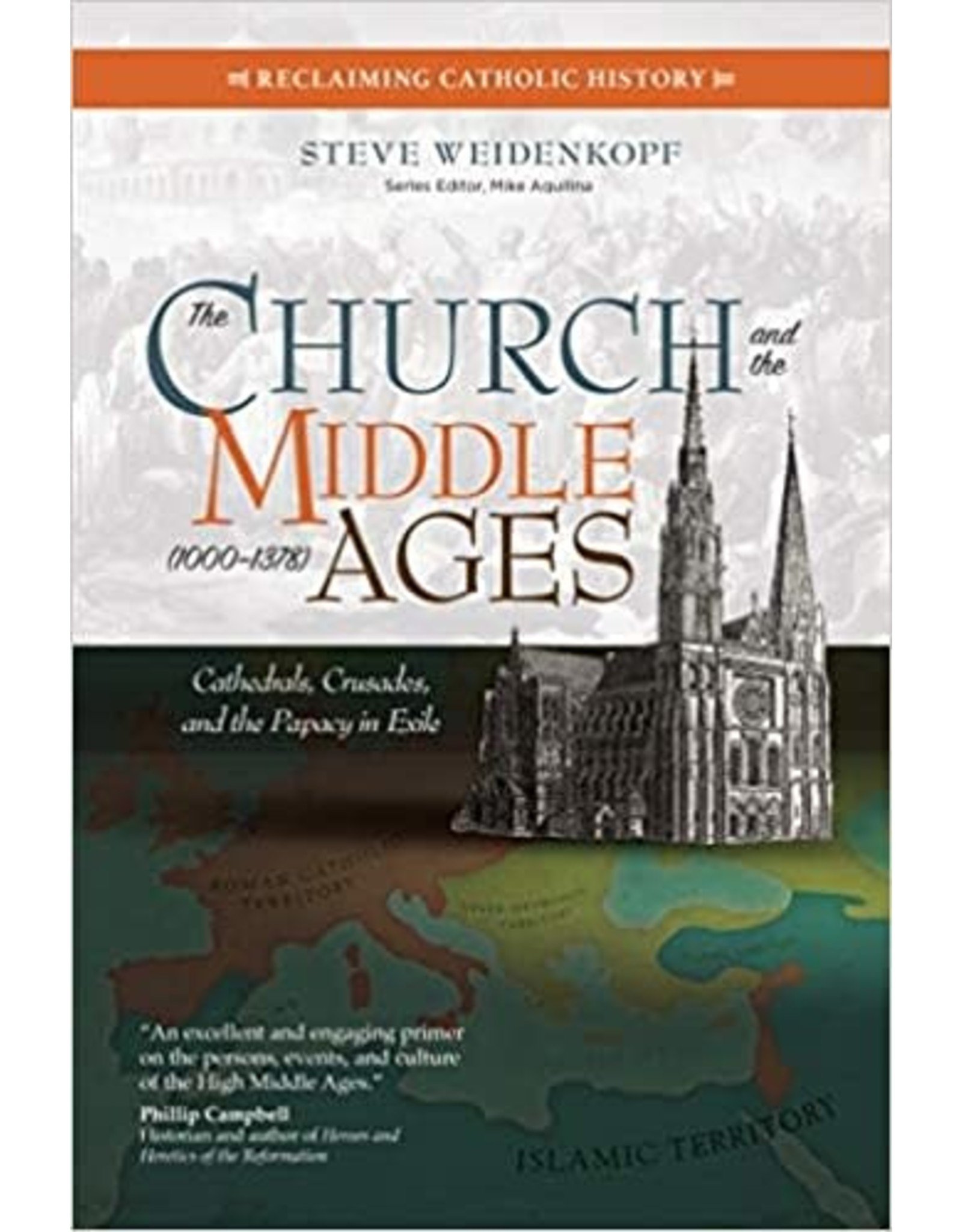The book cover titled "The Church and the Middle Ages, 1000 to 1378," authored by Steve Weidenkopf, features a visually detailed layout. At the very top, an orange band with white text reads "Reclaiming Catholic History." Below this band is the author's name, Steve Weidenkopf, prominently displayed. The main title, "The Church and the Middle Ages, 1000 to 1378," is centered and features a subtitle in smaller text beneath it, "Cathedrals, Crusades, and the Papacy in Exile," printed in teal and orange. The central image depicts a large cathedral with two tall steeples, rendered in black and white, superimposed on a simplistic, unadorned map of Europe. To the right of the cathedral image, the map includes a region labeled "Islamic Territory." Additionally, there is a review quote by Philip Campbell on the cover, although it is too small and blurry to read clearly. The series editor, Mike Aquilina, is also mentioned in smaller text below the author's name.